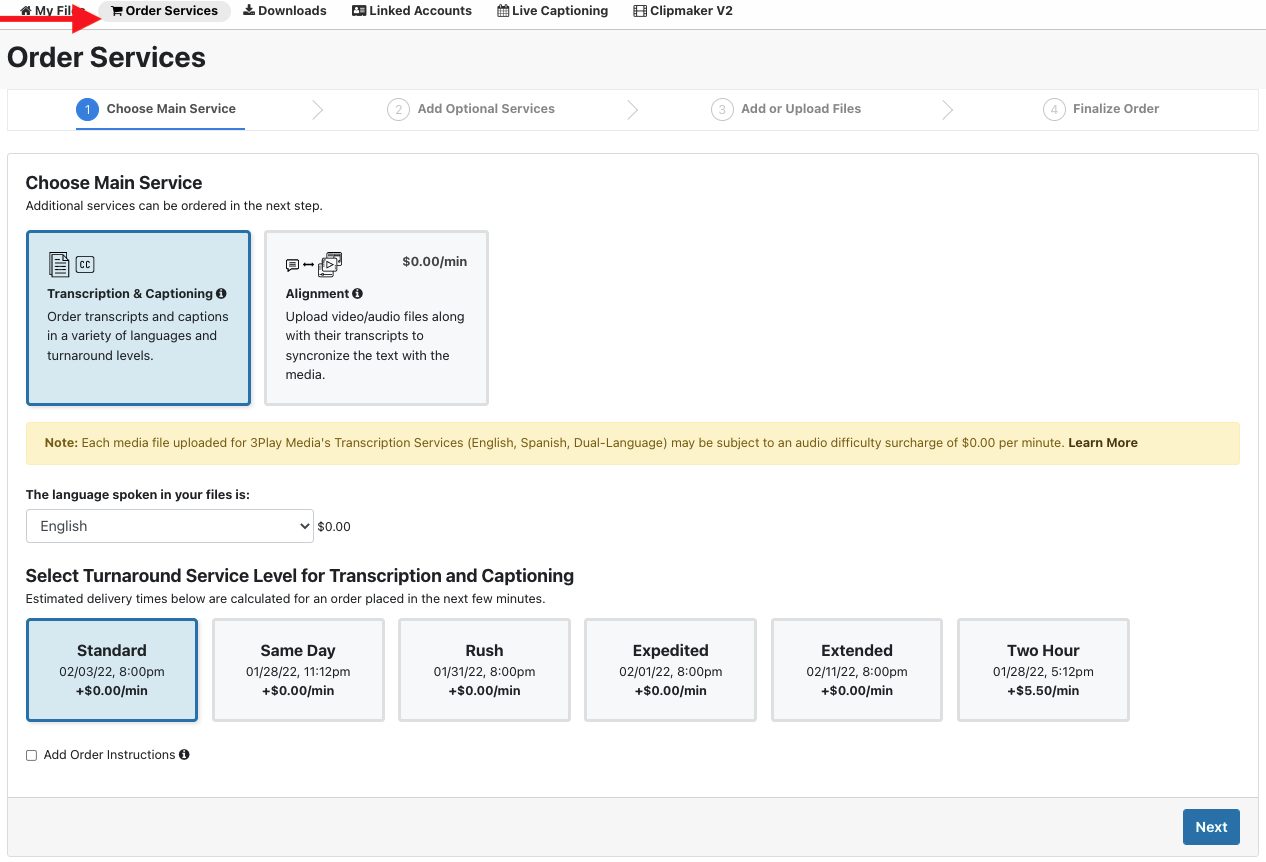**Detailed Caption:**

The image is a screenshot of a webpage, likely an order form for transcription services. The interface features a clean, predominantly white background with various sections and interactive elements that are organized in a structured manner.

At the very top of the page is a horizontal menu bar. From left to right, the first menu item is partially obscured by a red arrow (which appears to have been drawn in), with visible letters indicating it might say "My Files." Next to it are "Order Services," "Downloads," "Linked Accounts," "Live Captioning," and "Alaska's Clipmaker V2." Each menu item is paired with a small icon – for instance, "Live Captioning" features a calendar icon, "Downloads" has a download symbol, and "Order Services" shows a card. The "Order Services" button appears in gray, suggesting it is the currently active section.

Underneath this menu bar, the screen is divided into multiple sections focused on ordering transcription services. 

The first section, titled "Order Services," sports a blue circular icon with the number "1" and prompts the user to "Choose Main Service." Within this section, there are two options: "Transcription and Captioning" and "Alignment." The "Transcription and Captioning" option appears in blue, indicating it is currently selected, while the "Alignment" option is grayed out. Below this, a note in a yellow box provides additional information about file requirements.

Further down, another segment is dedicated to language selection, where it is indicated that the language spoken in the files is English, and the current selection count stands at zero.

The next section, labeled "Select Turnaround Services for Transcription and Captioning," offers various speeds of service completion. The options presented include "Standard," "Same Day," "Expedited," "Extended," and "Two-Hour." The "Standard" option is highlighted in blue, showing a completion time of 8 p.m. The other options are grayed out and currently all have a zero cost associated with them.

At the bottom right corner, there is a blue "Next" button poised for advancing to the next step of the ordering process.